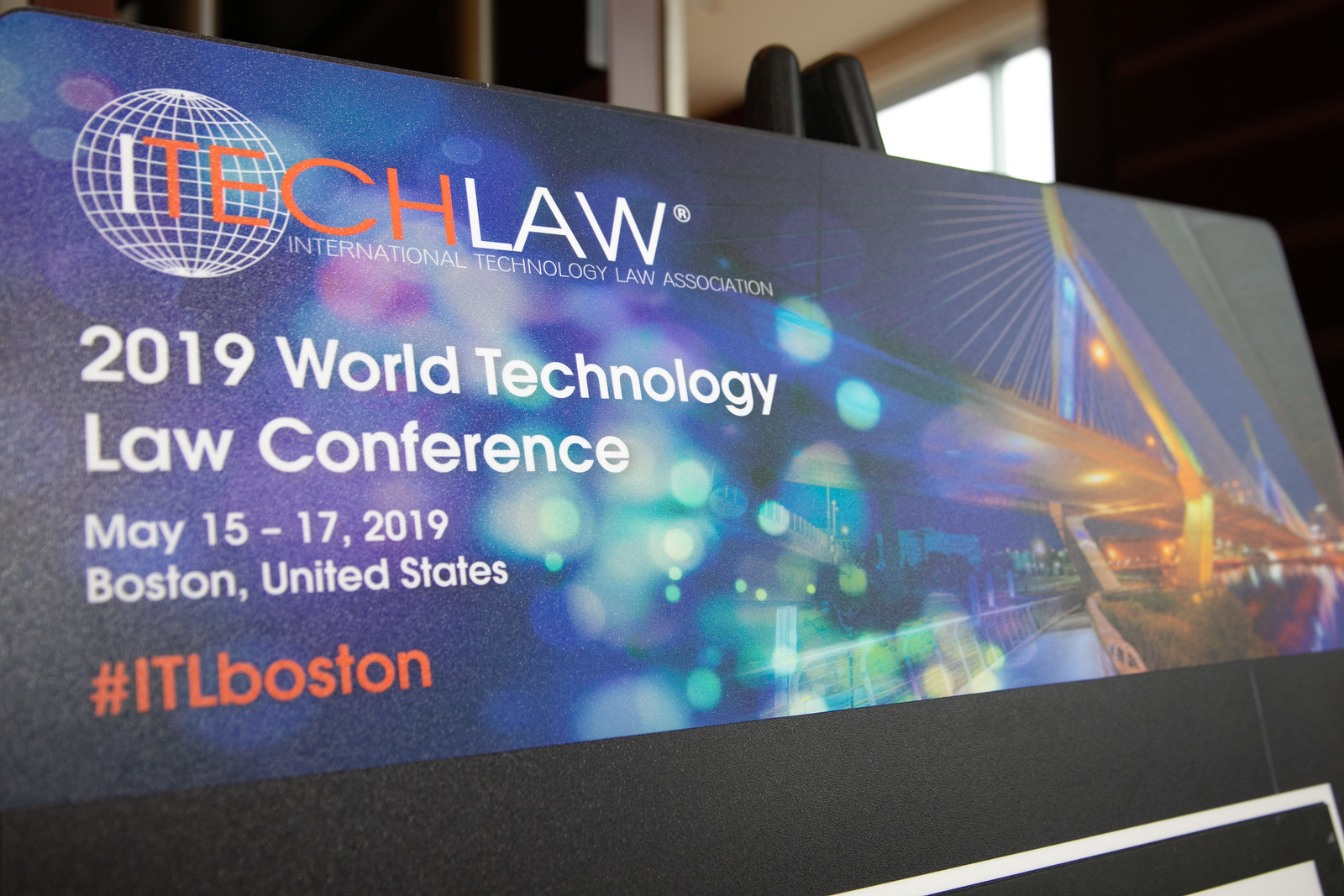The image depicts a detailed sign from the 2019 World Technology Law Conference. Located in the upper left corner, the logo features "iTech Law" prominently displayed, with "Tech" in orange and "Law" in white, followed by a trademark symbol. The logo is accompanied by a globe with intersecting lines. Beneath the logo, it reads "International Technology Law Association" in smaller capital letters. The main text on the left side of the sign announces "2019 World Technology Law Conference" in white bold letters, with the event dates "May 15th to 17th, 2019" and location "Boston, United States" prominently displayed. The bottom left corner features the hashtag "ITLBOSTON" in orange. On the right side of the sign, there is an image of a cityscape featuring a large bridge over a river, with glittering blue lights. The background includes black walls, a bright window allowing light to filter through, and a faintly visible beige ceiling.